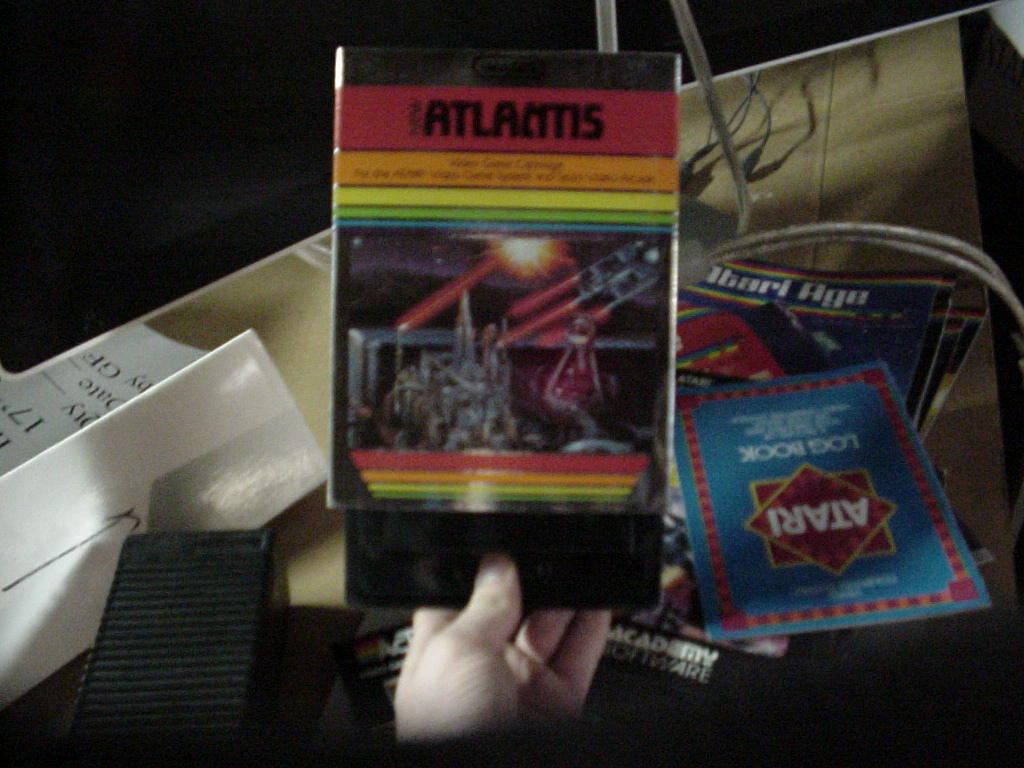A slightly blurry image captures a hand, presumably of a Caucasian individual, holding up a classic video game box titled "Atlantis." The front cover of the box features an illustration of a man piloting a sleek, silver space vehicle, flanked by a character on his right. In the background, a mountainous landscape stretches beneath a blue sky, where an object hurtles through the air, emitting a red flame. Scattered across the table surface behind the hand are several pamphlets branded with "Atari." Prominently, a blue pamphlet titled the "Atari Logbook" and another labeled "Atari Age" can be seen. Toward the bottom of the image, partially visible text starting with "ACT" hints at the logo for Activision, a well-known video game company. To the left of the hand, a rectangular black box likely represents a component of the gaming system, set against a light tan-colored table. Further left, a white box with indiscernible writing sits on the table, contributing to the nostalgic gaming tableau.